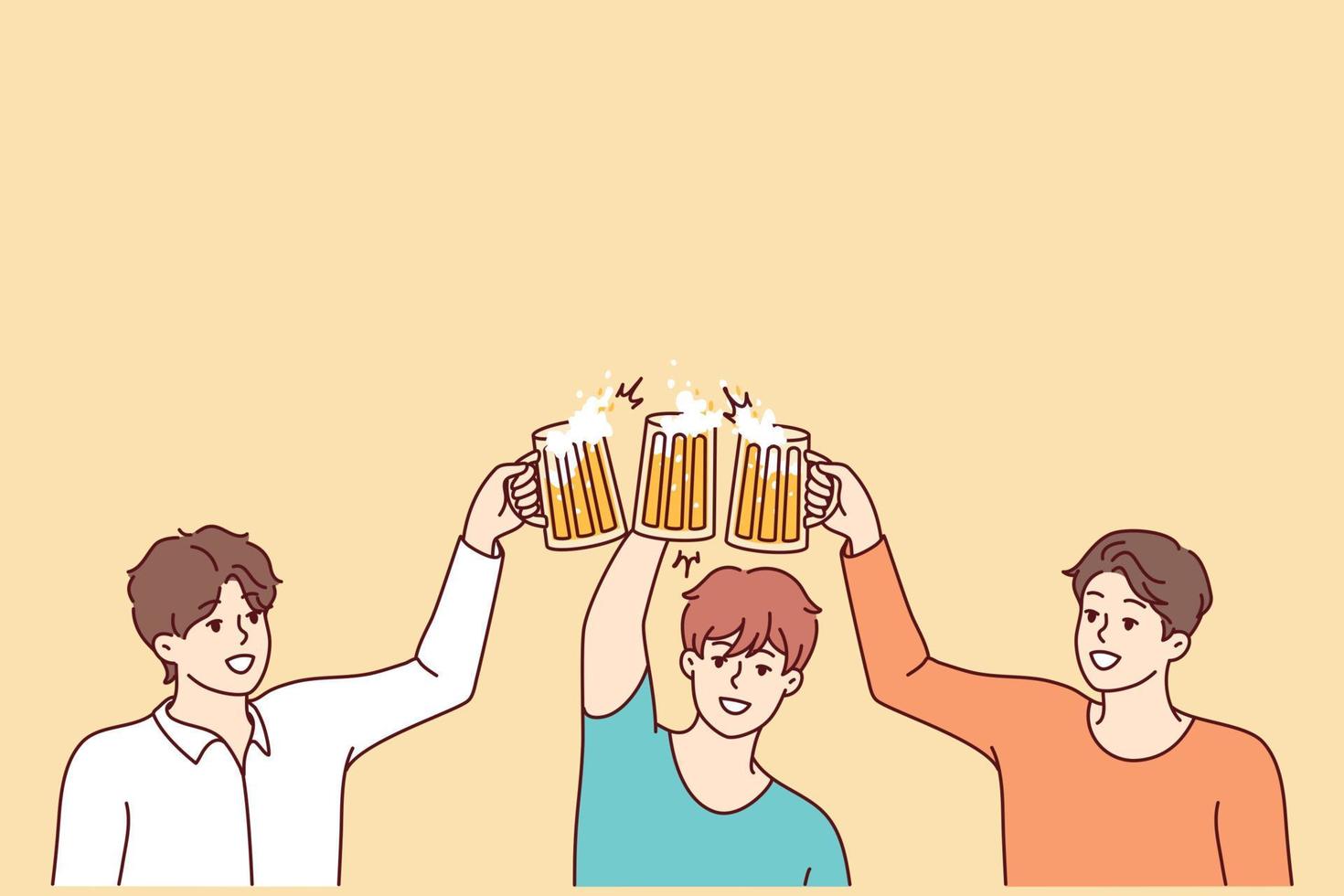This image is a digital or pen drawing featuring a minimalist depiction of three characters celebrating with beer. The background is entirely yellow, taking up the top half of the image while the bottom half is occupied by the trio. Each character holds up a mug of beer, depicted with a brownish hue and topped with white foam, as they clink their mugs together in a toast. 

The first character sports a white shirt and has brown hair. The second character is dressed in a blue shirt and has reddish-brown hair. The third character wears an orange shirt and also has brown hair. Facial features on these characters are simplistic, with dots and a small line for eyes and a black outline for the mouth, filled with white. Though their gender is not explicitly indicated by their features, their short hair may suggest they are male. The overall style is characterized by its lack of sharp details and an emphasis on a cheerful, lightweight atmosphere.